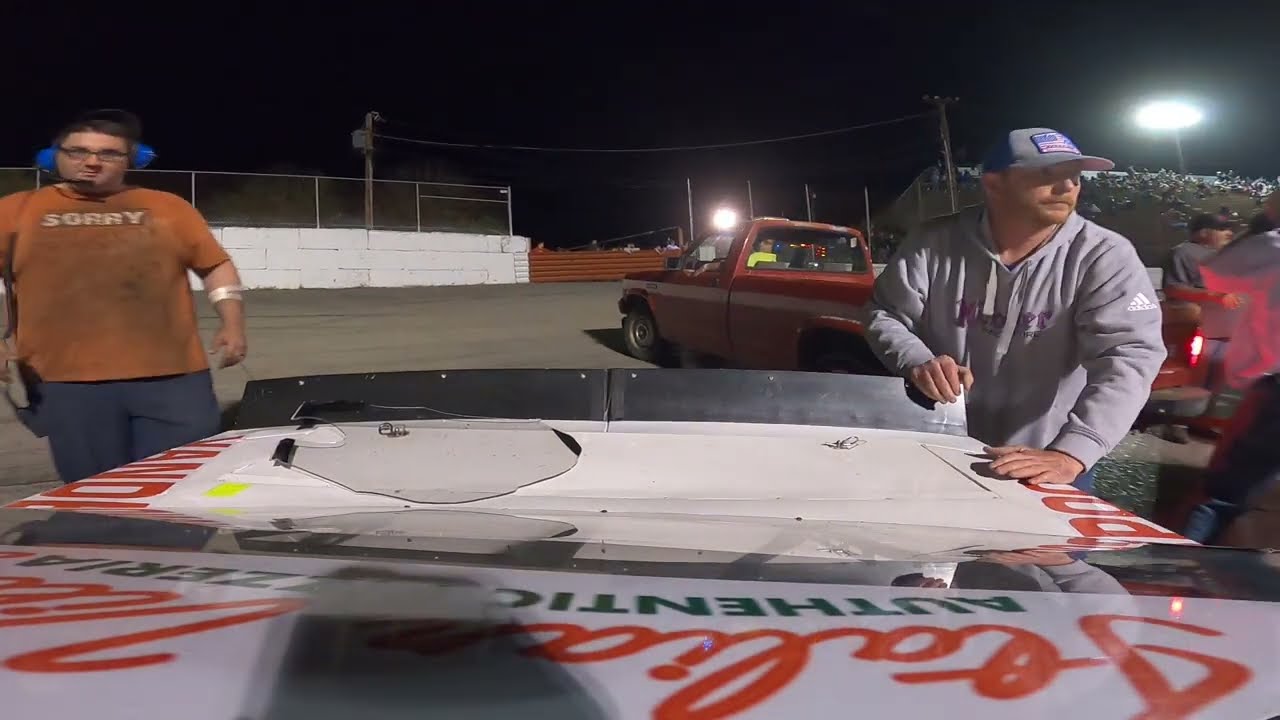This night-time outdoor photograph captures a bustling scene at a racetrack stadium, possibly around the pit stop area. The dark sky fills the top portion of the image, serving as a backdrop to the brightly lit activity below. Central to the image is the hood or possibly the trunk of a white vehicle, adorned with red cursive print that's difficult to decipher and green block letters spelling out "authentic."

On the left side of the vehicle stands a man clad in a dirtied short-sleeved orange t-shirt with white lettering that reads "sorry." He is equipped with over-the-ear blue headphones with an attached mic and is dressed in black pants. A white armband encircles his left arm, and he sports a goatee, black glasses, and dark hair.

To the right of the vehicle, another man leans forward, seemingly exerting an effort to push it. He is dressed in a light gray hooded sweatshirt, known as a hoodie, and a gray ball cap. His attention appears directed to the side, perhaps focused on an unseen task or person.

Behind the men, the racetrack's white concrete wall and fencing are visible. Further in the background to the right, a set of bleachers filled with spectators can be seen, along with a grassy hillside. A red pickup truck is prominently parked facing away from the viewer.

Illumination from a floodlight in the upper right corner adds to the dynamic atmosphere of this scene, lending clarity to the intricate details and interplay of light and shadow.